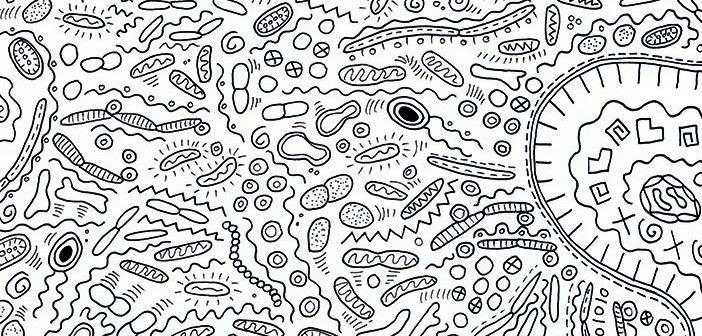The image is a black and white, hand-drawn depiction, resembling a wallpaper or intricate pattern, on a stark white background. The drawing is composed of various bacteria-like and germ-like forms rendered in varying thicknesses of black lines, reminiscent of ink or felt pen. These oblong, rectangle, and circular shapes feature diverse internal designs, some having squiggly lines, zigzags, or segmented interiors that evoke the appearance of cells and their organs. The detailed drawing includes abstract representations such as circles within circles, spirals, X's, and rectangular shapes. Some shapes are detailed like suns with rays, worms with stripes, and gear-like objects. To the right, there appears to be a track-like formation, packed with different shapes such as a continuously looping circle, crosses, and open squares. The overall image is densely packed with these varied, detailed designs, creating a crowded and intricate visual.